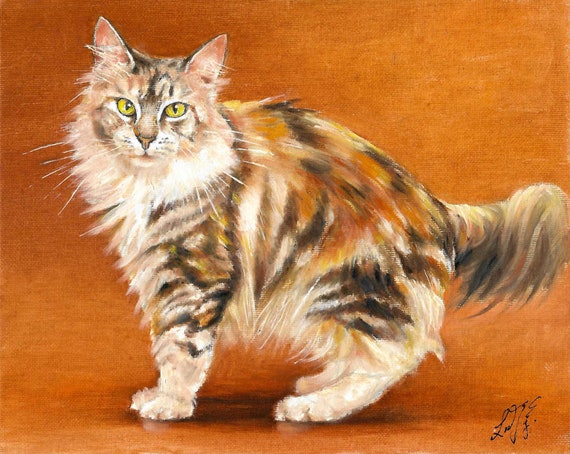This vibrant painting captures a long-haired, fluffy cat in exquisite detail, set against a dynamic, thatched orange backdrop that transitions from darker to lighter shades. The cat, adorned with tiger-esque markings in browny black, oranges, yellows, and patches of light tan and white, stands in a natural pose with its back feet touching the ground and its body slightly upward, suggesting movement into a sitting position. It has a long, curving furry tail and is facing to the left, with its head turned to gaze directly at the viewer, creating an impression of soulful connection. The cat's striking golden-green eyes, pointed ears with tufted tips, and bright white whiskers add to its expressive demeanor. The artist meticulously detailed the varied textures and colors of the cat’s fur, and incorporated shadows underneath, enhancing the painting’s realism. The piece features the artist's cursive signature in the bottom right-hand corner, completing this rich and detailed composition.